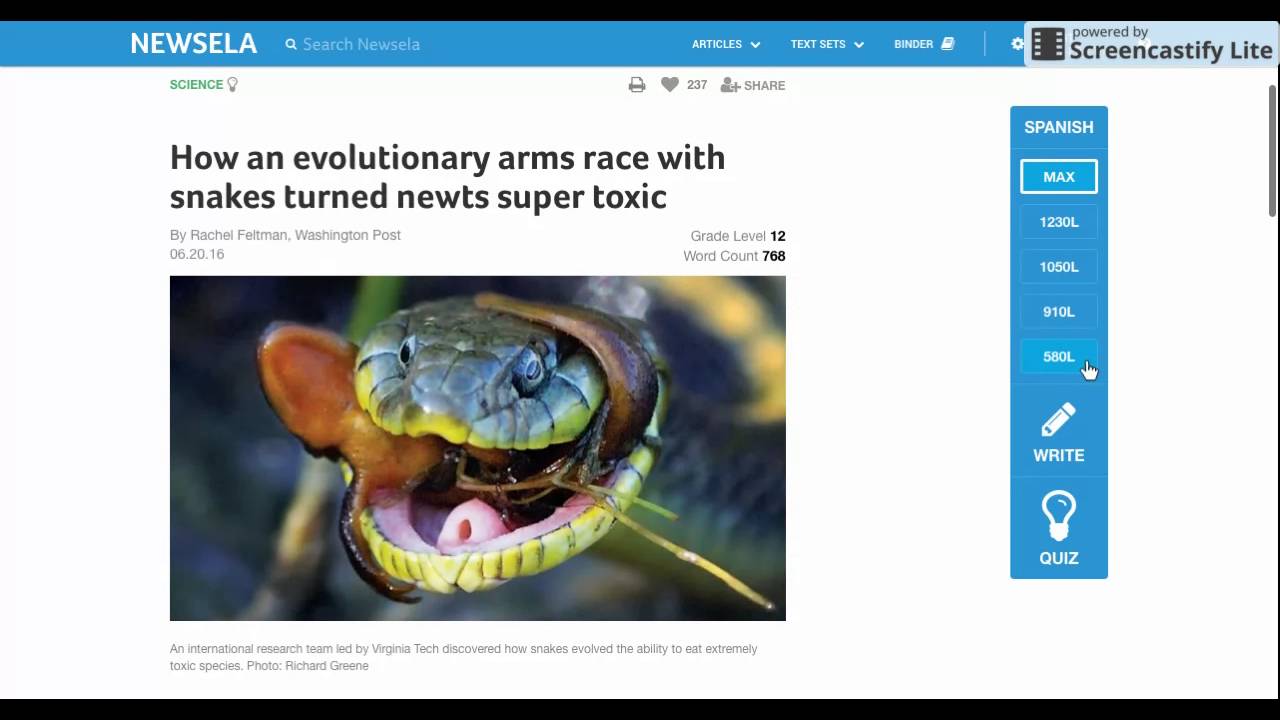The screenshot displays the Newsela platform, prominently featuring the search bar and options like Articles, Text Sets, and Binder. At the top right corner, there is a "Powered by Screencastify" icon along with a lightbulb icon. The main screen is themed around "Science," and includes various interactive elements such as a printer icon, a heart icon with a count of 237, and a share button.

On the right-hand sidebar, there are options for selecting the Spanish language and different text complexity levels, outlined in rectangles: Max, 1230L, 1050L, 910L, and 580L. Below these options, there are buttons labeled "Write" accompanied by a pencil icon, and "Quiz" signified by a lightbulb icon.

The article displayed is titled "How an Evolutionary Arms Race with Snakes Turned Newts Super Toxic," authored by Rachel Feltman of the Washington Post. It is designated for a 12th-grade reading level, spanning 768 words, and was published on June 20, 2016. There is also a vivid image of an open-mouthed snake accompanying the article, enhancing the engaging layout of the page.